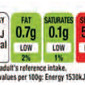This image showcases a partial view of a nutritional information label, typically found on the side of a food product packaging. The focus is on four rounded rectangles displaying various nutritional values. The first rectangle on the left is white and partially cut off, making its content unreadable. Adjacent to it is a green rectangle indicating "Fat: 0.7g, Low, 2%". The following green rectangle states "Saturates: 0.1g, Low, 1%". To the right, there's a partially visible red rectangle, with its content cut off and unreadable. Below the rectangles, there is some text, partially obscured, that mentions "Adults' Reference Intake Values per 100 grams" and an energy value of either "150" or "1538 K". The image provides an incomplete but insightful glimpse into the nutritional composition of an unspecified food item.